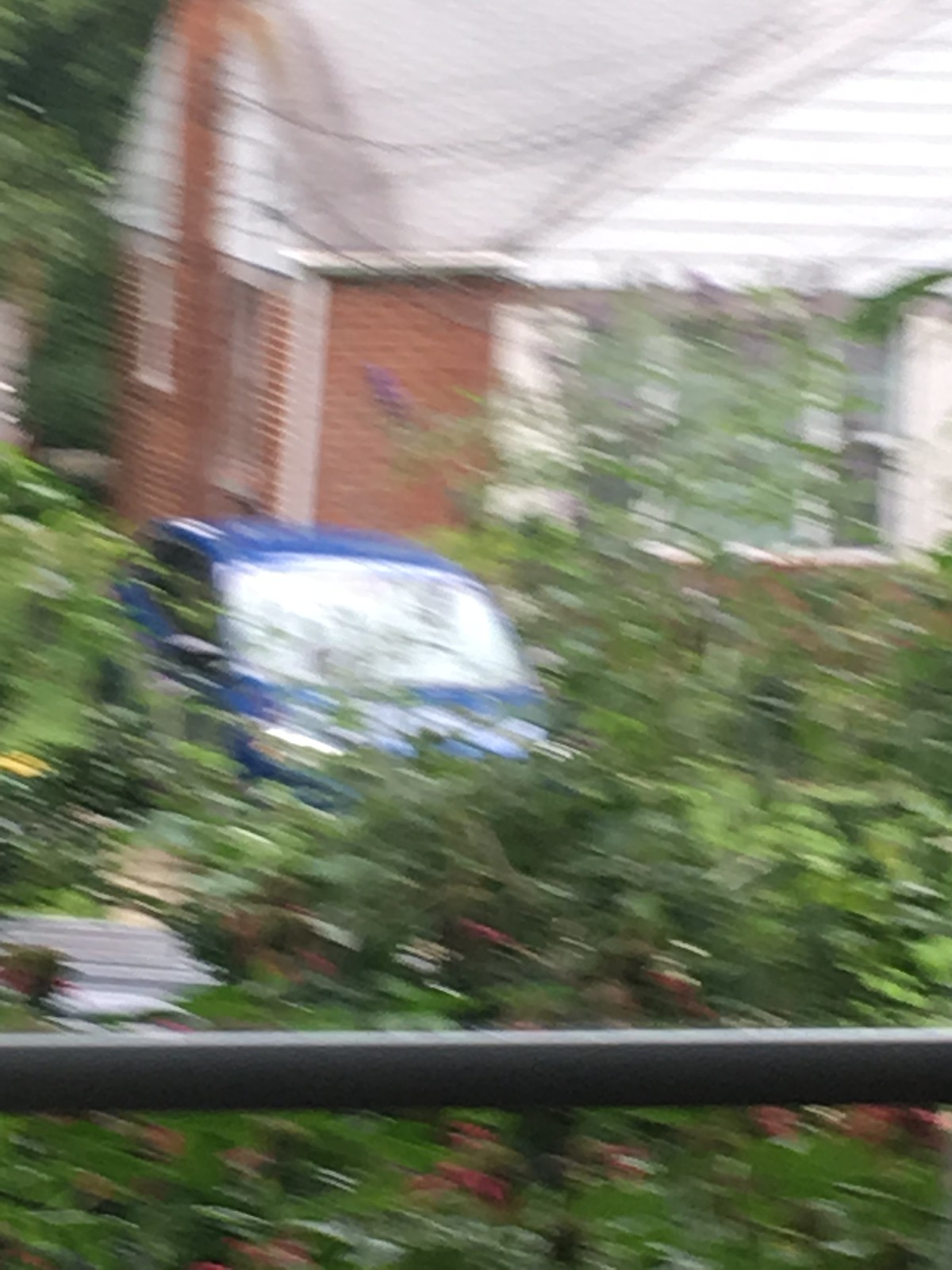In this slightly blurry outdoor photograph, the perspective of the photographer is from behind a black horizontal bar that stretches across the lower part of the image. Beyond this bar, dense greenery, predominantly bushes with an abundance of leaves, occupies about half of the frame, forming a natural screen. Peeking through the foliage in the background is the front section of a small blue vehicle, showcasing its windshield and hood while leaving the rear portion obscured and indeterminate. Behind the vehicle stands a red brick two-story house, adding a residential backdrop to the scene. The overall composition, though unclear, suggests a tranquil suburban setting with elements of nature and architecture intertwined.